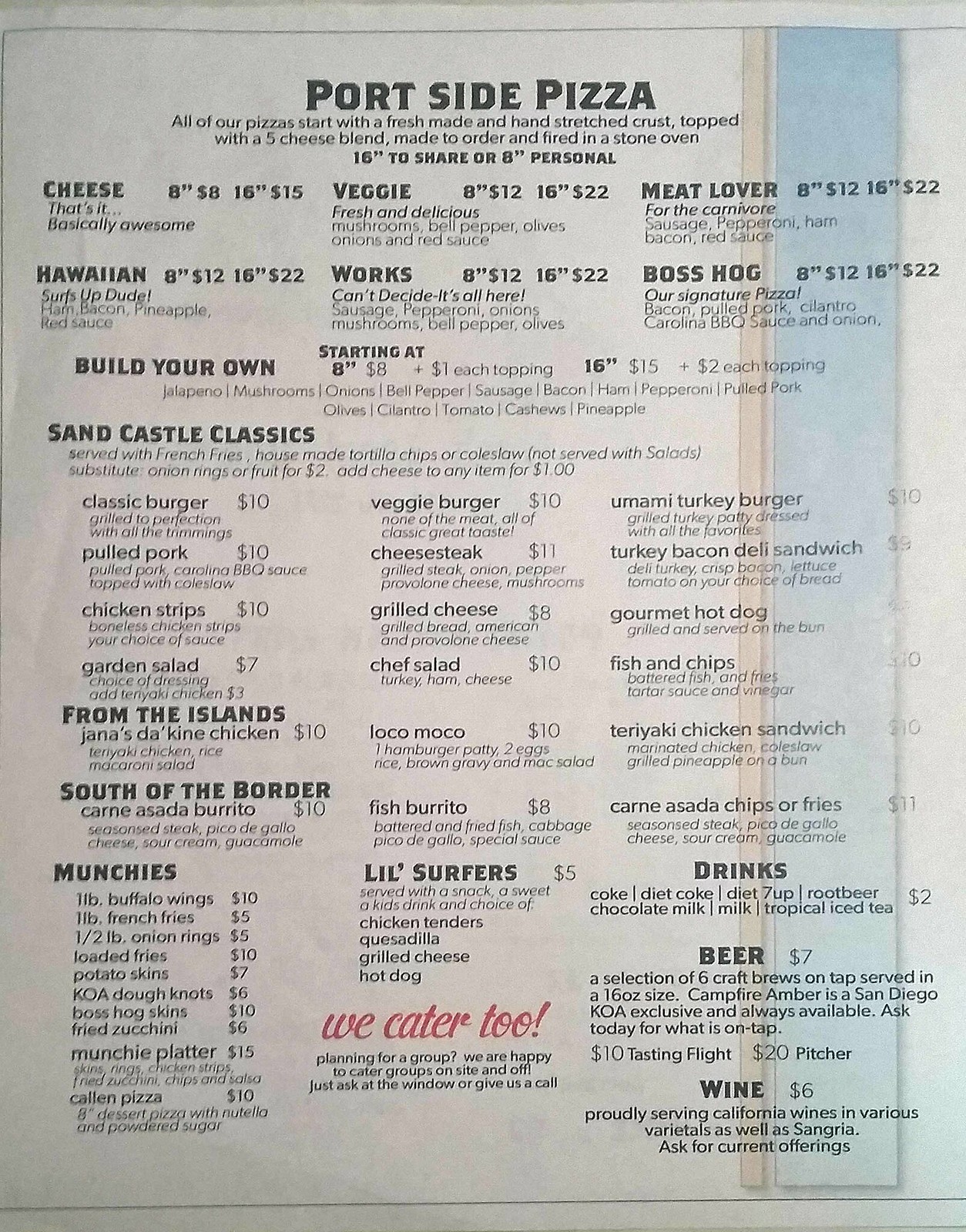The image showcases the menu of Port Side Pizza, printed on white paper and placed against a white background. The menu has a distinct layout characterized by a white stripe along the right edge, followed by a pale blue stripe approximately an inch wide, and a narrow brown stripe further to the left. At the bottom, a black line indicates the printing limits.

At the top of the menu, in bold, uppercase letters, is the restaurant name, "PORT SIDE PIZZA." Beneath it, a description in smaller font reads: "All of our pizzas start with a fresh-made and hand-stretched crust, topped with a five-cheese blend, made to order and fired in a stone oven. A 16-inch to share or 8-inch personal."

The pizza options are listed with brief descriptions:
- Cheese: It's basically awesome.
- Veggie: Fresh and delicious.
- Meat Lovers: For the carnivore.
- Hawaiian: Serves up, dude.
- Works: Can't decide? It's all here.
- Boss Hog: Our original, our signature pizza.

Additional lines of text provide prices for different sizes and the option to build your own pizza with starting prices.

Further down, the menu features "Sandcastle Classics," which are served with French fries, house-made tortilla chips, or coleslaw, but not with salads. There's an option to substitute onion rings or fruit for $2, and to add cheese to any item for $1. Classic items include:
- Classic Burger
- Pulled Pork
- Chicken Strips
- Garden Salad
- Veggie Burger
- Cheese Steak
- Grilled Cheese
- Chef Salad
- Loco Moco
- Fresh Burrito
- Umami Turkey Burger
- Turkey Bacon Deli Sandwich
- Gourmet Hot Dog
- Fish and Chips
- Teriyaki Chicken Sandwich
- Carne Asada Chips or Fries

The menu also contains categories like "From the Islands," "South of the Border," "Munchies," "Little Surfers," "Drinks," and "Beer and Wine."

Prominently displayed in the middle of the menu, in red cursive writing, is the phrase "We cater to!" followed by an exclamation mark. Below it, in black text: "Planning for a group? We are happy to cater groups on-site and off. Just ask at the window or give us a call."